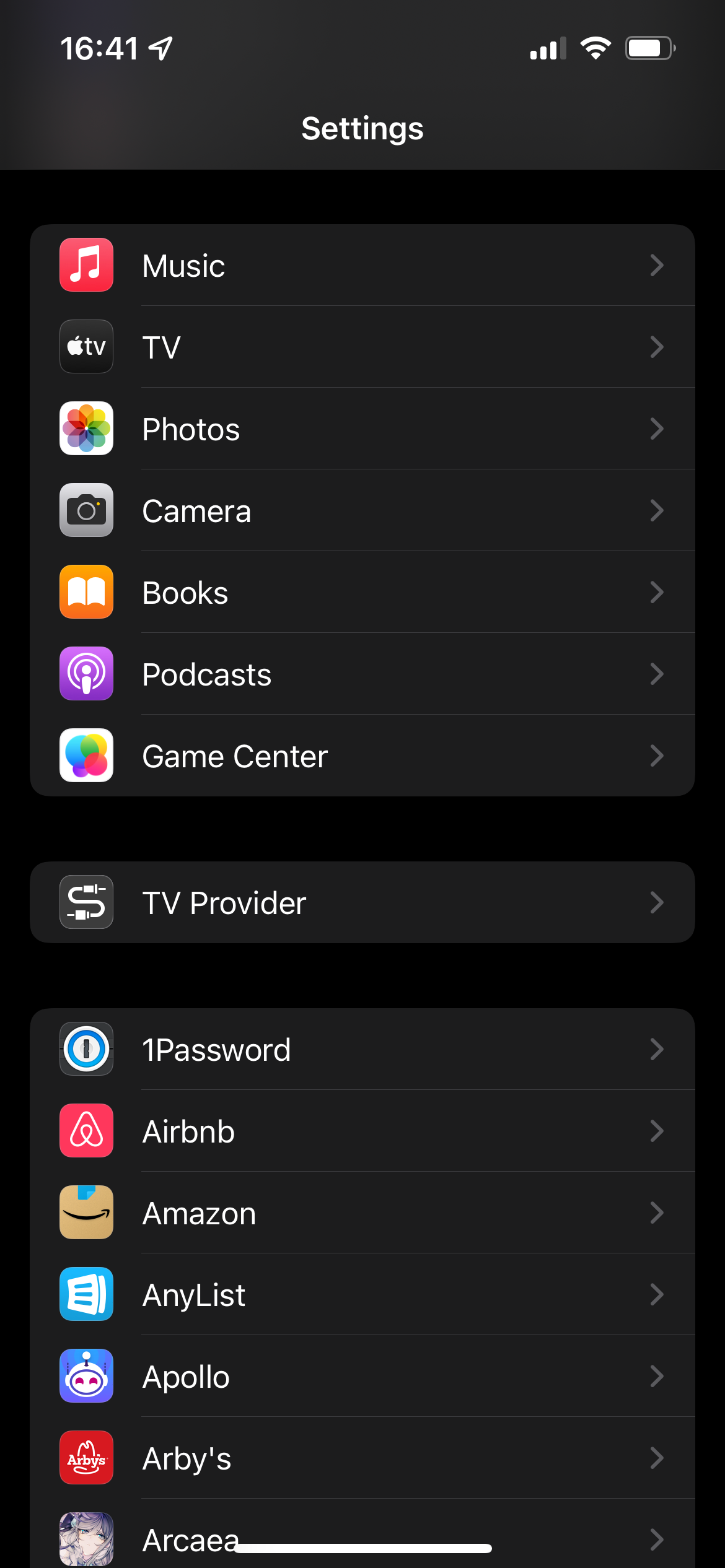This is a settings screenshot from a cell phone displaying three distinct sections. The background is black, while each section is highlighted in a lighter shade of black, and the top bar bears the word "Settings" in white. 

**First Section:**
There are seven items listed vertically, each accompanied by a left-aligned icon:
1. **Music**
2. **TV** (icon resembles an Apple TV)
3. **Photos**
4. **Camera**
5. **Books**
6. **Podcasts**
7. **Game Center**

**Second Section:**
A single option is listed:
- **TV Provider**

**Third Section:**
Seven more options are displayed, each prefixed with an icon:
1. **1Password**
2. **Airbnb**
3. **Amazon**
4. **AnyList**

The image conveys a structured layout of settings on a black-themed interface, emphasizing the hierarchical organization and ease of navigation through distinct categories.